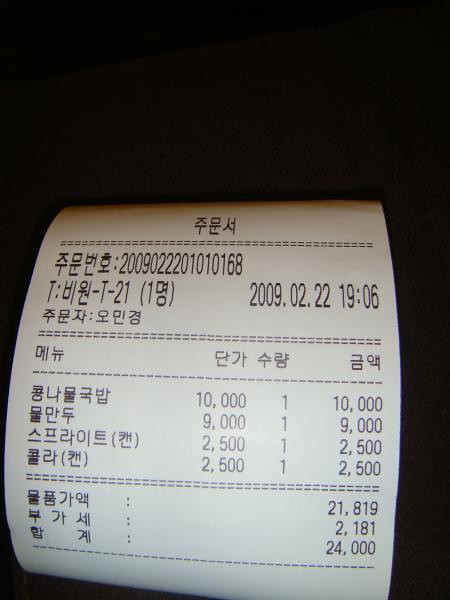The image features a curled receipt, with the top edge of the paper bending slightly outward. The black background suggests that the photograph was taken at night, although the camera flash has illuminated the white paper of the receipt effectively. Text on the receipt is printed in an Asian language, likely Taiwanese, given its distinct script.